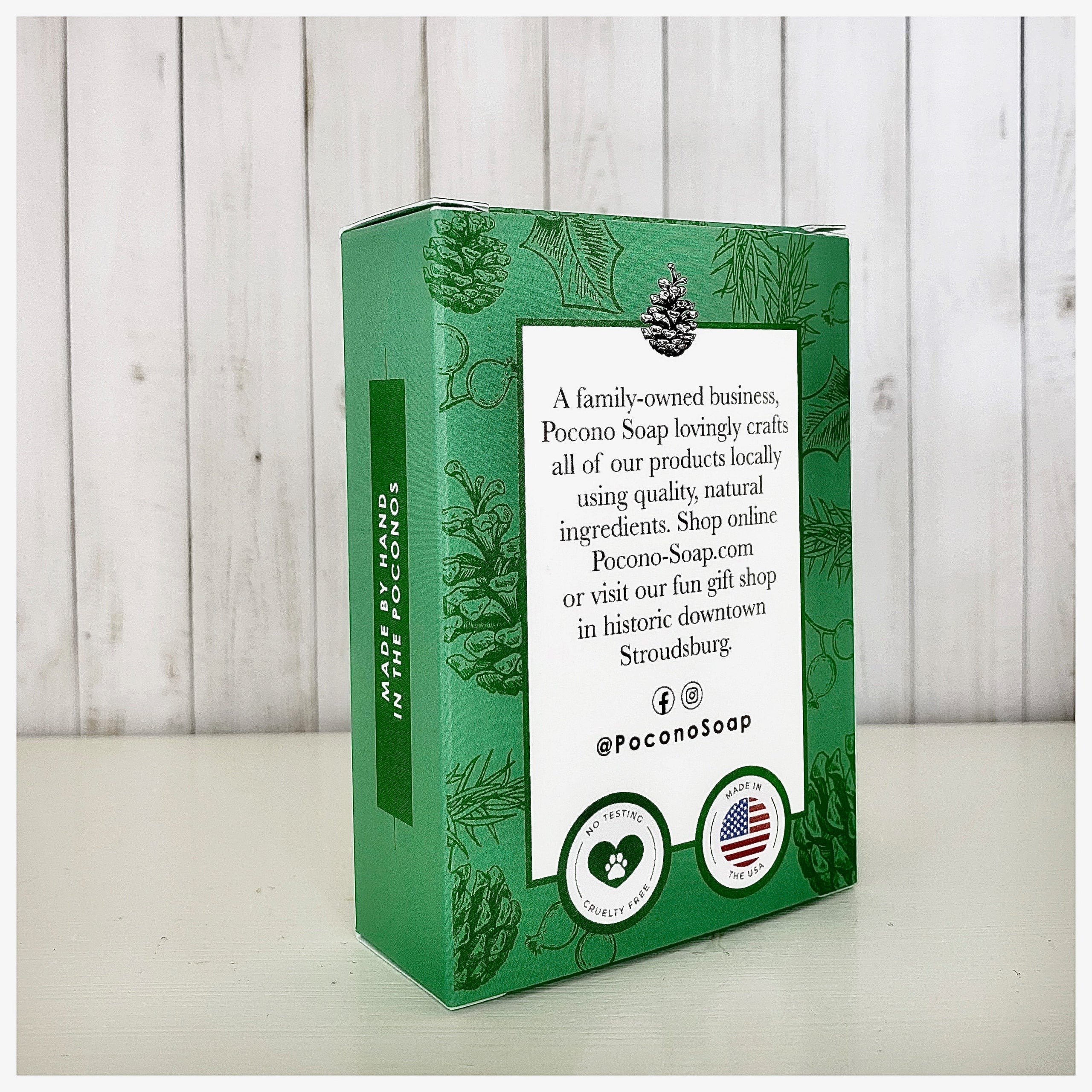The image is a detailed color photograph capturing a green box, reminiscent of sage green, set vertically on a cream-colored surface with a white, vertical plank-board backdrop. The box features intricate artwork of pine cones and leaves sketched around its green border. Central to the box is a white panel containing an image of a black and white pine cone along with black text. The text highlights that the product is crafted by the family-owned Pocono Soap, emphasizing the use of quality, natural ingredients, and inviting viewers to shop online at PoconoSoap.com or visit their lively gift shop in historic downtown Stroudsburg. At the bottom of this white panel are social media icons tagged with #PoconoSoap, followed by two circles: the left circle showcases a green heart with a paw print symbolizing cruelty-free, no animal testing practices, while the right circle displays the American flag, indicating the product is made in the USA. Additionally, the side of the box has the wording "Made by Hand in the Pocono" in white. The photographic style is representational realism, focusing on the intricate details of the product packaging.